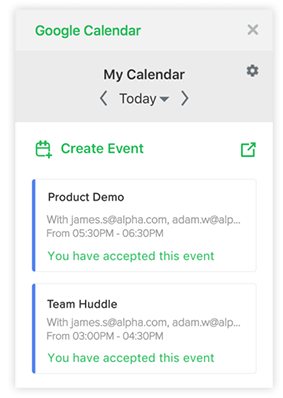The image features a clean white background with a gray bar at the top. In the middle of the bar, "Google Calendar" is prominently displayed in green. To the right of this, "My Calendar" is listed in green as well. Adjacent to these titles is a pair of brackets shaped like an arrow, and buttons for "Today" and a dropdown menu are positioned nearby. A settings icon is also visible. Below, the option to "Create Event" is marked in green.

Underneath, the calendar view highlights a scheduled event. A black text entry denotes a "Product Demo" with participants listed as "james.s at alpha.com" and "adam.w at alp..." The event is set from 5:30 PM to 6:30 PM, and a green text indicates that "You have accepted this event." To the left, there's a distinctive blue rectangle.

Further down, another blue rectangle marks the entry for a "Team Huddle" with the same participants, running from 3:00 PM to 4:30 PM. This event is similarly confirmed with a green "You have accepted this event" text.